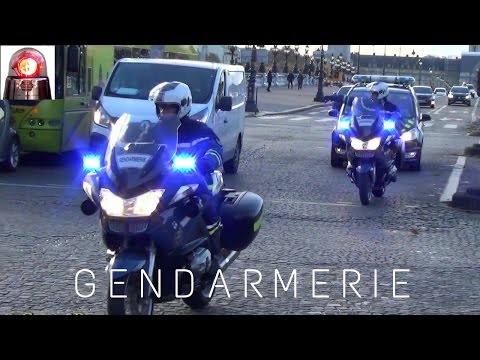The photograph captures a police motorcade navigating a cobblestone street, visible in its rectangular shape with distinctive black borders at the top and bottom. The word 'Gendarmerie' overlays the bottom black band in thin, white, capitalized letters, signifying a law enforcement presence, likely from another country. Dominating the left side of the image, a blue motorcycle with a lit blue siren is driven by a helmeted officer in a black suit. A similar motorcycle follows slightly behind and to the right, also sporting blue lights. Ahead of these motorcycles are multiple vehicles, varying in color from blue to light gray or white, including a conspicuous flat top square vehicle on the left. Additional vehicles are scattered in the background, suggesting an urban setting though buildings are not prominent. In the top left corner, a white square houses a conical siren light—metal-based with a clear plastic dome encasing a red light. Some greenery is barely discernible on the very left, and street posts or lamp posts stand in the background. The street features multiple white lines, hinting at a crosswalk further back.